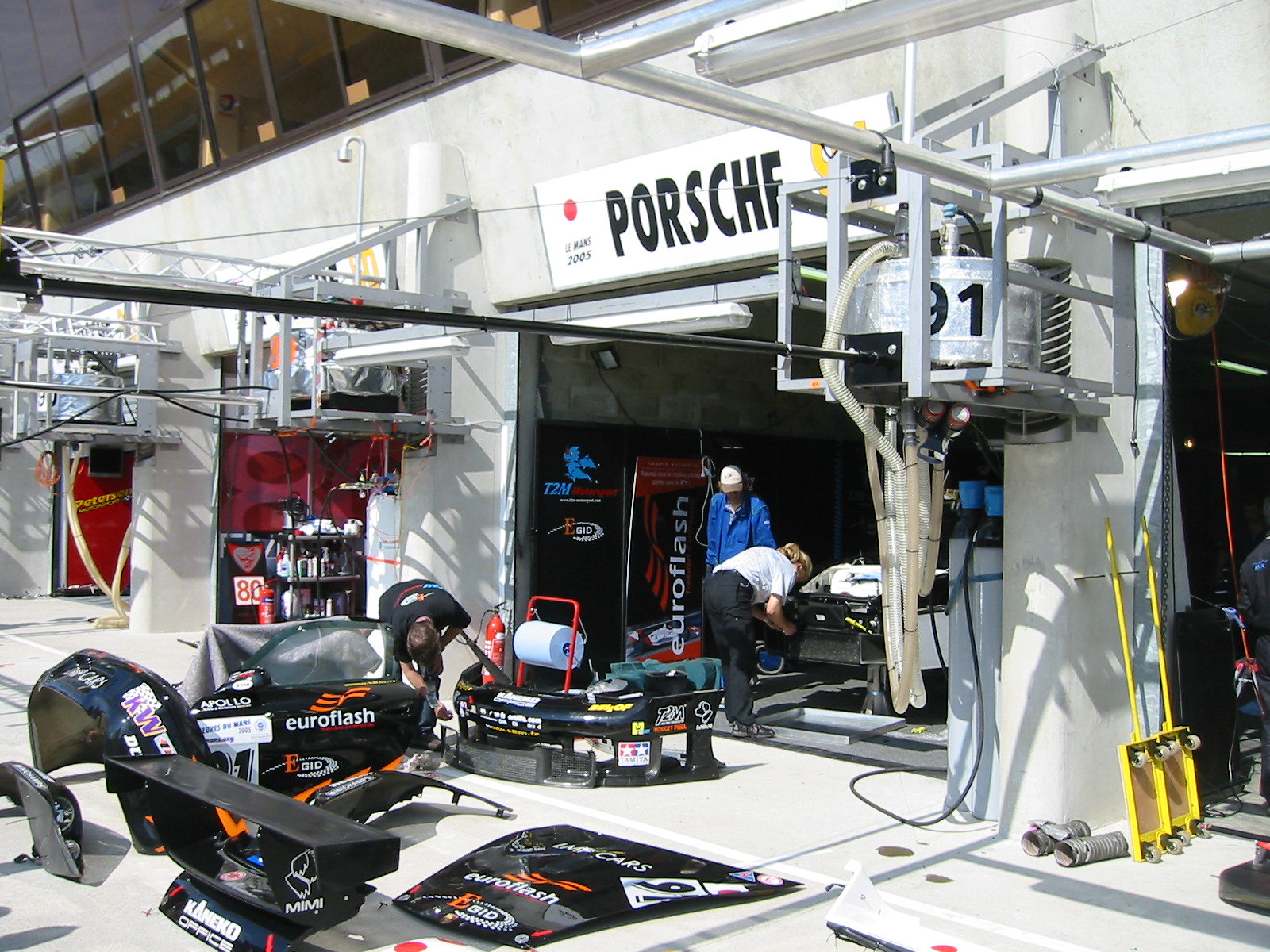This is a detailed color photograph taken indoors at what appears to be a garage area of a racetrack, likely a car repair shop or a Porsche racing crew station. The walls and floor are gray, giving an industrial look to the environment. Dominating the scene is a large white sign with a red ball on the left and a yellow design on the right, and the word "Porsche" prominently printed in bold black letters in the center. 

In the foreground, there are two individuals working on car parts scattered around—one is wearing a hat and a blue jacket, standing and looking down at another person who is bent over, dressed in dark pants and a light shirt. On the far lower right, a yellow handheld cart or lift is visible. 

The background reveals further details, including a partially disassembled Porsche with a front hood displaying the number 91 and a visible number 80 in another area. Additionally, black items labeled with "Euroflash" in white and orange designs are scattered around. A row of windows high up on the walls floods the area with light. Two notable elements are a soda machine inside the left wall and shelves stocked with cans and parts, indicating further activity and equipment storage. Garages from other manufacturers are also visible further down, suggesting a hub of automotive activity.

Overall, the scene is vibrant with mechanical activity, reflecting a busy environment where vehicles are meticulously taken apart and repaired.